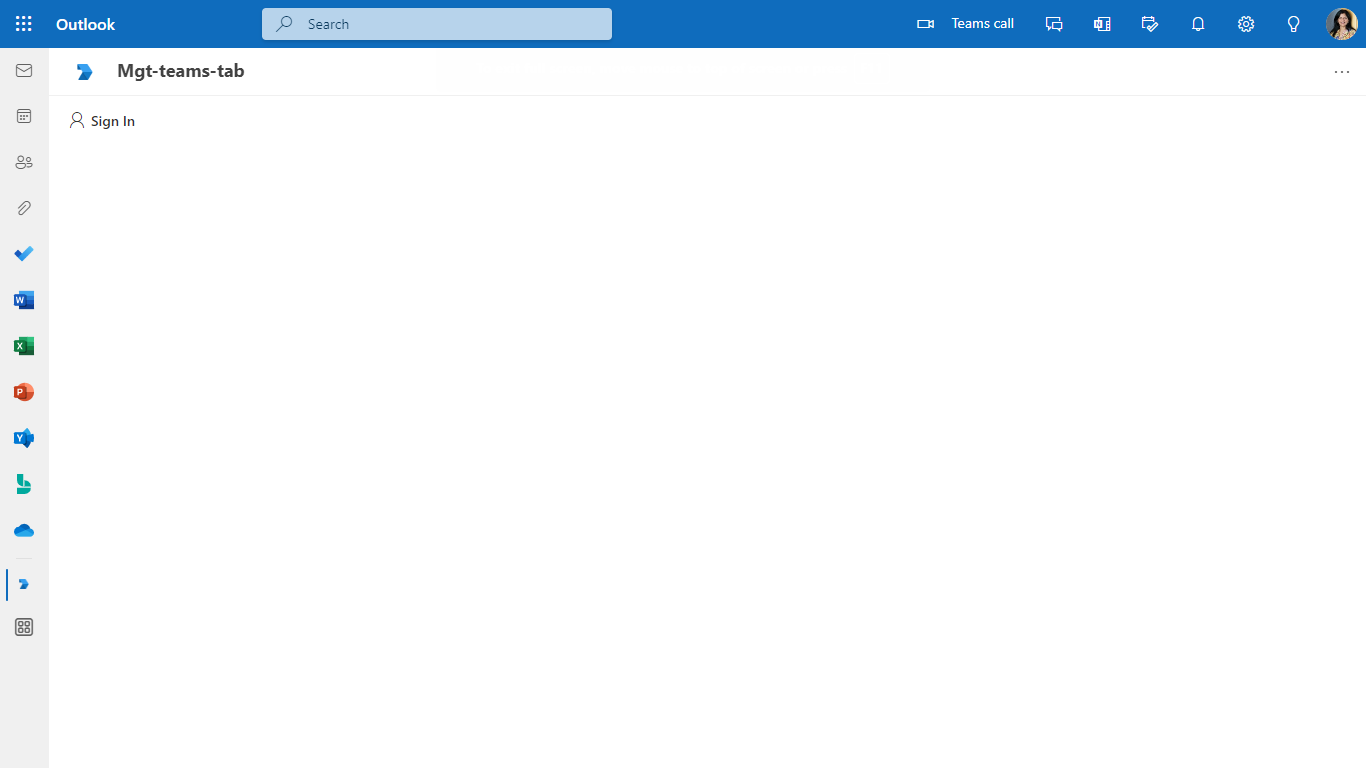In the screenshot of Outlook, the interface is vividly detailed, starting with the top left corner where a square-shaped icon composed of three rows of three dots each can be seen. This icon is followed by the bold, white text "Outlook" displayed on a prominent blue header bar. Adjacent to "Outlook" is a search bar featuring a magnifying glass icon and the word "Search" inside it.

Moving right, there are several icons in sequence: first, the Teams call icon, followed by a conversation icon. Next come two additional icons whose specifics are less clear. These are succeeded by a bell icon for notifications, a settings gear icon, and a light bulb icon for insights or tips. Finally, at the far right end of the header bar, there is a profile picture representing the user of the screen.

Under this header, in the leftmost column, multiple icons depict various functionalities. Starting from the top, the icons likely represent Mail, Calendar, People, Attachments, Tasks (with a checkmark symbol), Word, Excel, and several other apps or features, indicative of commonly used Microsoft Office and Outlook tools.

On the upper right-hand corner of the interface, there is a tab labeled "Management Team" that appears to offer sign-in functionalities or access to specific management features.

This detailed layout shows a comprehensive view of the Outlook interface with various tools and resources at the user’s disposal.